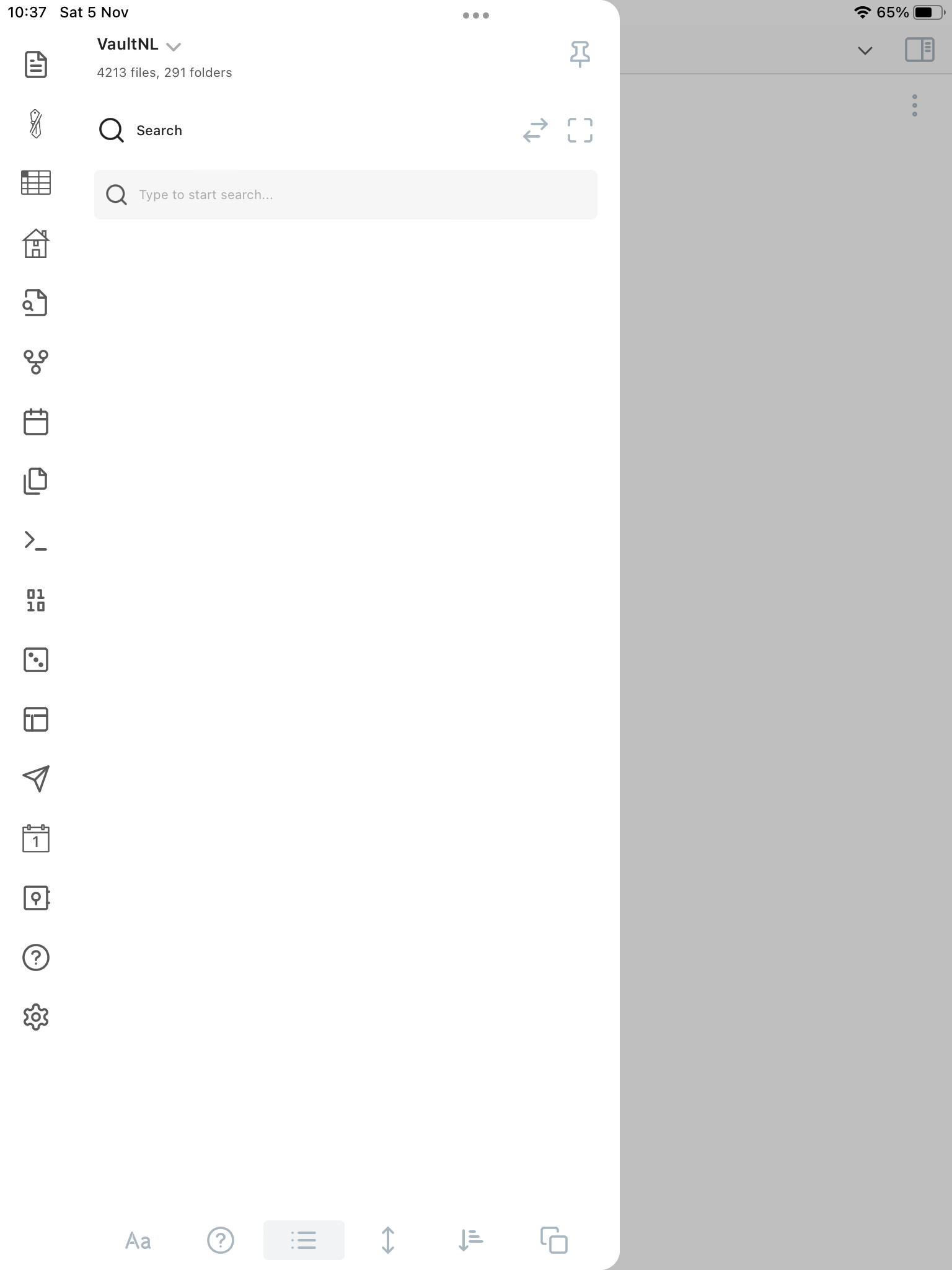The image depicts a software interface with a predominantly white background and minimal text. On the left side of the screen, a vertically aligned pane features various buttons, likely related to programming, networking, and general settings, suggesting that this is an IT or software development tool. The central section of the page is mostly blank white space. An overlay, titled "Vault NL," appears after a side pane is clicked, displaying a search bar with no additional content visible. The interface's color scheme primarily uses black for any icons or text. Additionally, the image includes details about the user's device status, showing a 65% battery level and strong Wi-Fi connectivity. Formatting tools, such as options for capitalization, paragraph formatting, and bullet points, are visible at the bottom of the interface.